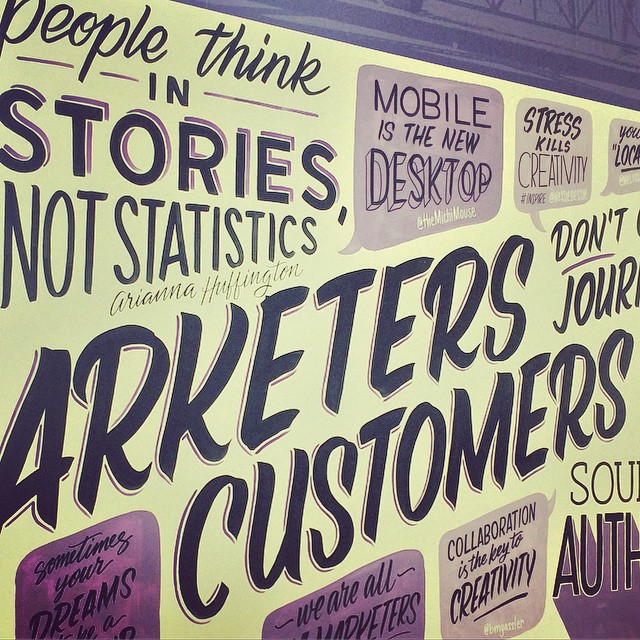This image features a bold, inspiring sign on a yellow background with a mix of black and purple text. Predominantly, the text reads, "People think in stories, not statistics," attributed to Arianna Huffington in cursive letters. Below this, three purple dialog boxes add extra quotes: "Mobile is the new desktop," "Stress kills creativity," and partially visible text starting with "You" and "L-O-C-A," suggesting something cut off. Centered on the sign is a fragmented message that appears to say, "Architeers don't like customers," with the phrase continuing to, "Sometimes your dreams. We are all collaboration is the key to creativity." Each of these quotes has a social media handle beneath it, making it easy to look up the authors online. The design uses varied fonts and styles, enhancing the visual engagement.